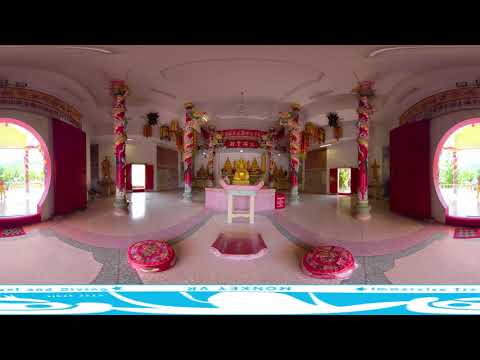The image depicts a brightly lit, large indoor space that appears to be a shrine or possibly a highly decorated room within a home or store. The predominant color scheme consists of various shades of pink, ranging from hot pink to softer hues, enriched with red and golden accents. The room features a pink ceiling, a pink floor that has gray undertones, and hot pink walls adorned with intricate gold and floral decorations.

At the top of the image, four large hot pink columns are visible, each wrapped with flowery decorations spiraling down. In the center of the background wall, there are golden statues that resemble Buddhist monks or figures typically found in a monastery, hinting at an Asian cultural influence.

There are two large, circular windows or possibly round entryways, one on the left and the other on the right, allowing natural daylight to flood the room. On the floor, two seat cushions are positioned for seating. The overall brightness, intricate floral decorations, and the traditional Asian elements contribute to a serene and sacred atmosphere within the space.